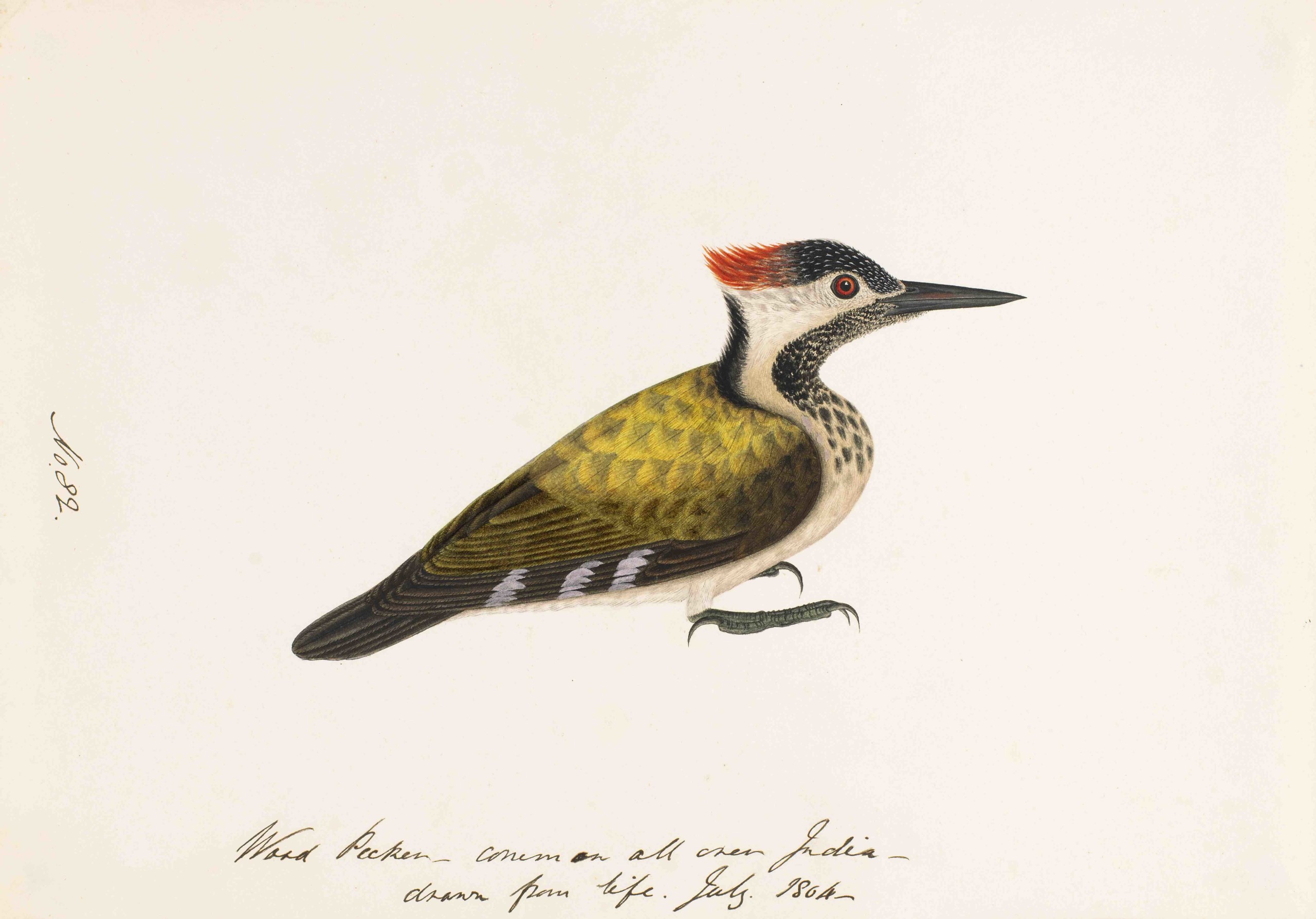This illustration, set against an off-white background, depicts a woodpecker with vibrant, detailed artistry. The bird features an olive green plumage that darkens towards the wing tips, a white belly, and a black and speckled chest. Its face presents a mix of black and white speckling, and it prominently displays a small but vivid red crest at the back of its head. The woodpecker's eye is a dark reddish-brown, while its beak is long and black, contributing to its distinctive appearance. Additional details include its short, dark blackish-brown tail and black feet. Handwritten in cursive beneath the bird are the words: "woodpecker, Common all over India, drawn from life, July 1804." The annotation “number 82” can be seen to the left of the bird.